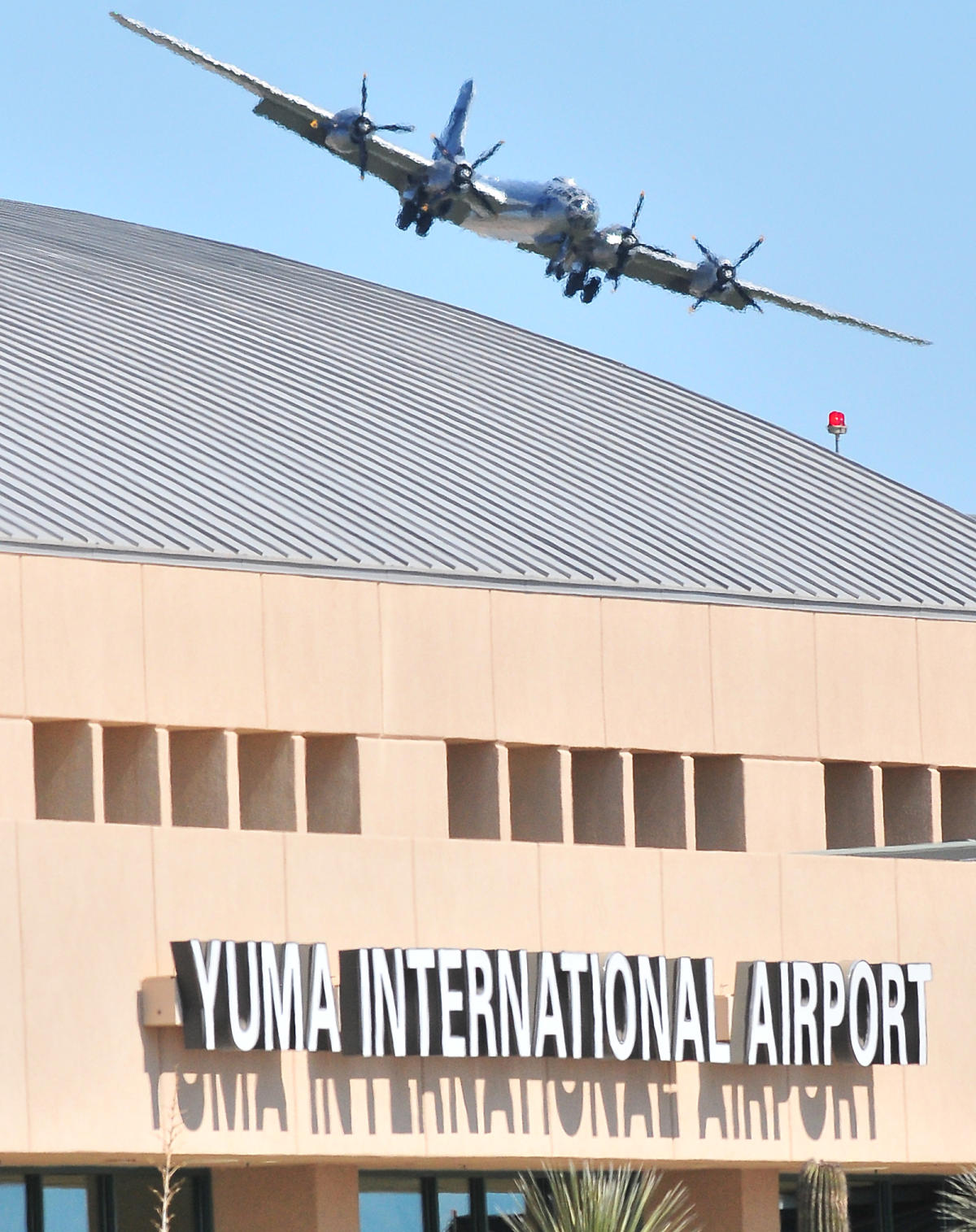The photograph captures the large, tan hangar-like building of Yuma International Airport, prominently featuring a sign in white letters that cast shadows underneath, suggesting a high sun. The building’s facade resembles adobe design, accented by a light gray, steel roof with raised ridges. Above the roof, a four-engined, silver aircraft with its wheels down is seen descending at an angle, appearing close but in the background, poised as if about to land. The airport's architecture includes pillars with an open-air bottom layer and groups of five windows along the top. In the foreground, a distinct red warning light reminiscent of an old police siren stands on the right side of the roof. The top of a cactus and other plants are just visible under the sign, adding a touch of local flora to the scene. The entire setting is bathed in natural daylight under a clear blue sky.